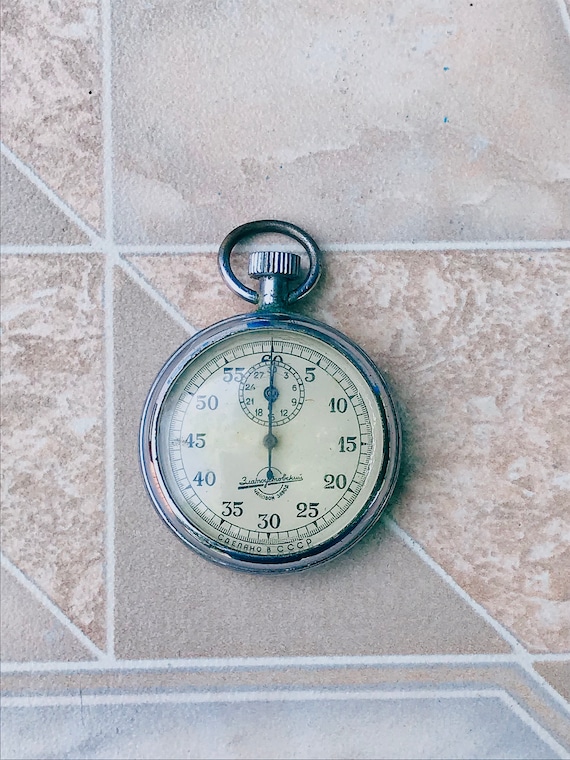This color photograph features an antique stopwatch, estimated to be around 50 to 60 years old, placed on a backdrop of gray and white tile that resembles stone with linear sections and a mix of gray and brownish swirls, suggesting a granite surface. The stopwatch has a silver or metal outline and a slightly worn appearance, with a winding adjustment knob and a circular ring at the top, which could be used to attach the stopwatch to a belt. The face of the stopwatch is protected by glass and displays time in increments of 5, marked as 5, 10, 15, 20, 25, 30, 35, 40, 45, 50, 55, and 60. Additionally, it features a smaller dial at the middle top with increments of 3, ranging from 3 to 30. The hands of the stopwatch are set at the 60 position. A group of Cyrillic letters is inscribed at the bottom of the stopwatch. This simple yet detailed timepiece captures the essence of a bygone era.